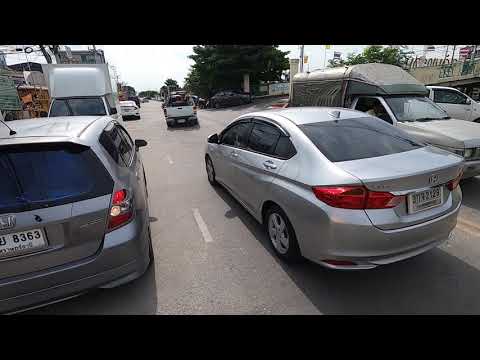The image captures a daytime scene on a busy road, seemingly outside the United States, as the observed traffic is driving on the left side. Prominently in the foreground are a gray SUV and a silver Honda Coupe moving forward. Preceding them, a white truck, a white van, and a white sedan can be seen heading in the same direction. On the opposite side of the road, a truck and another car drive in the opposite direction, separated by a yellow divider line. The background reveals a mix of makeshift buildings and business signs, with a large green tree adding some natural contrast. A strip mall is visible to the right, with parked vehicles including a camper trailer. The clarity of the scene suggests a clear day, with some direct sunlight casting shadows despite an otherwise overcast sky.